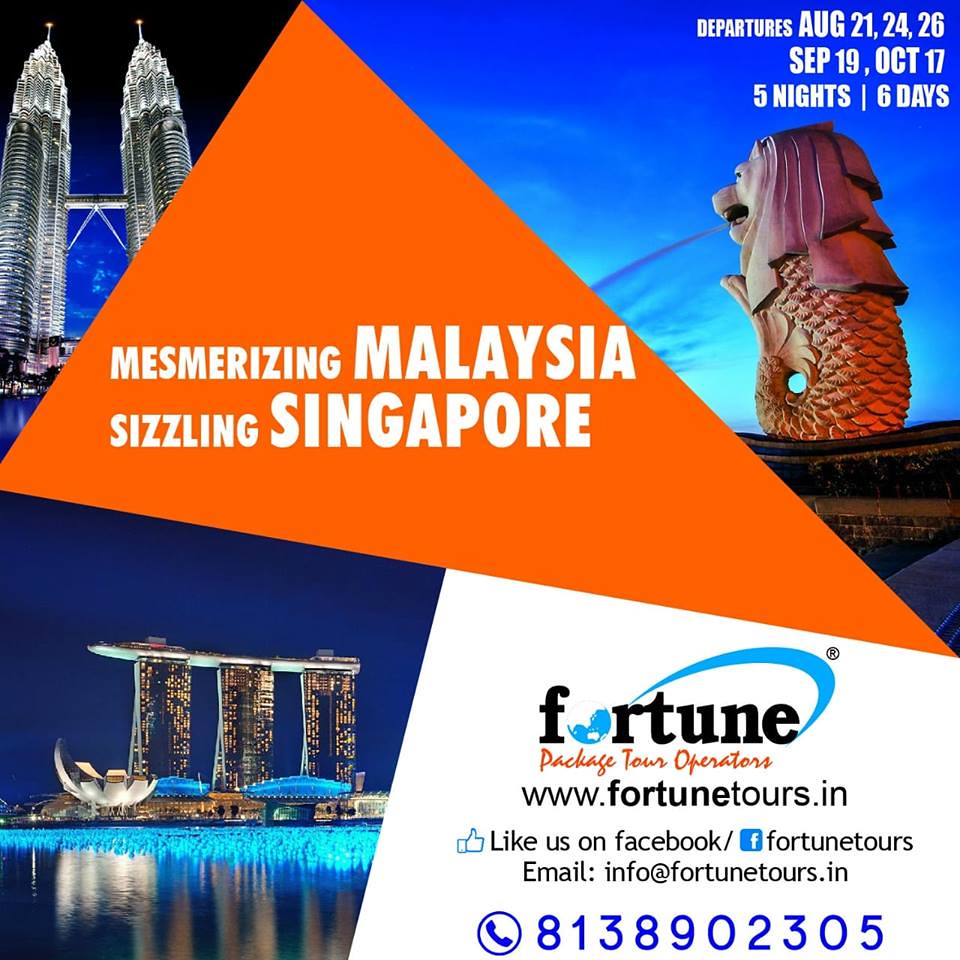This captivating travel advertisement by Fortune Tours showcases awe-inspiring destinations in Malaysia and Singapore with vivid imagery and alluring details. The top left photograph features a pair of matching skyscrapers connected by a walkway, their pointed tops adorned with lightning rods. To the right, a striking sculpture combining a lion's head and a fish's body catches the eye. The bottom left image displays three skyscrapers capped by an extended walkway, with additional buildings and water visible below. The central section of the poster, encased in an orange triangle, highlights the enticing call-to-action with white text reading "Mesmerizing Malaysia" and "Sizzling Singapore." The promotion offers packages for five nights and six days with departure dates on August 21st, 24th, and 26th, as well as September 19th and October 17th. Prominently displayed contact information directs potential travelers to the Fortune Tours website (www.fortunetours.in), encourages Facebook engagement, and provides an email (info@fortunetours.in) and phone number (813-890-2305) for inquiries.